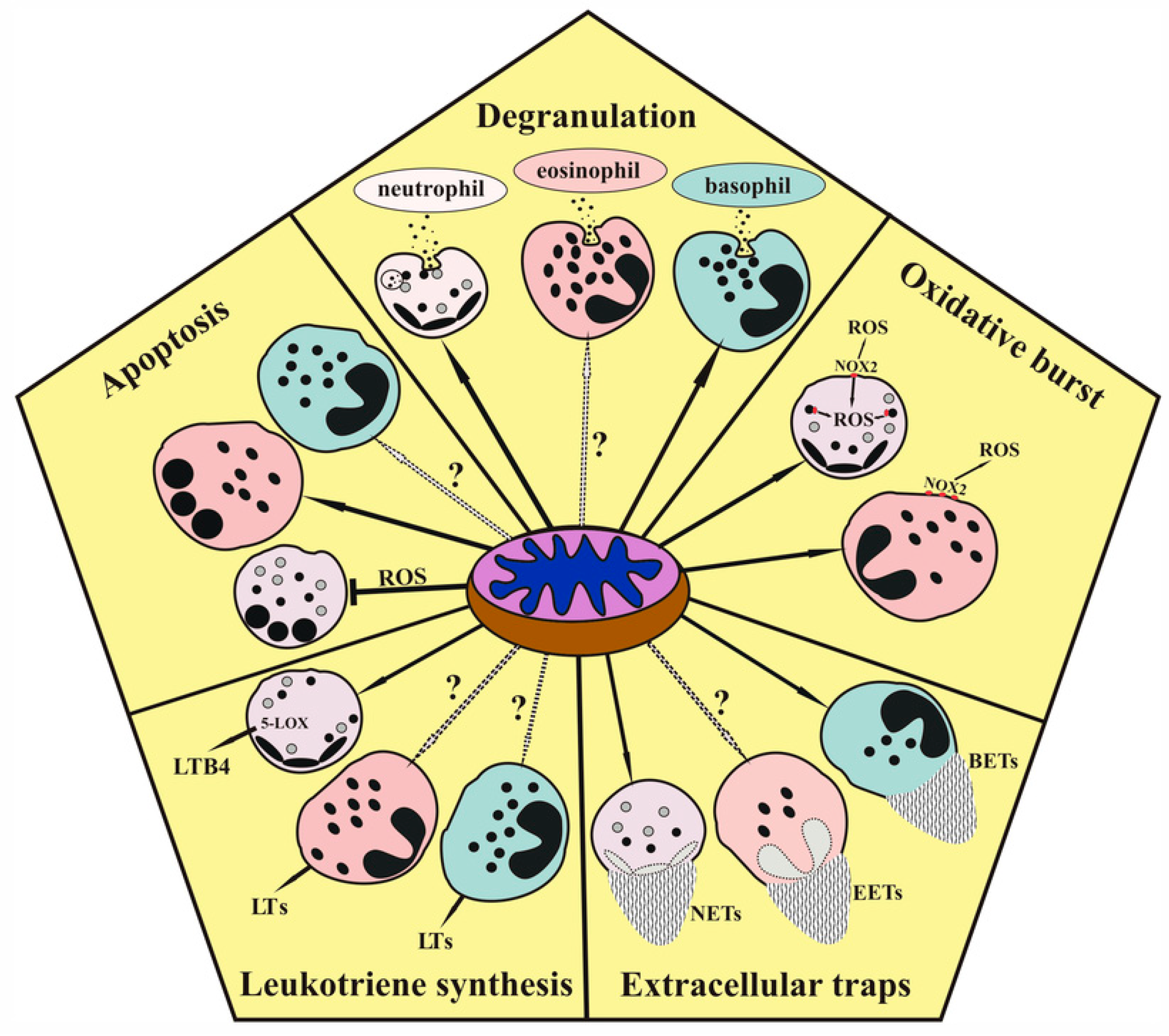The image showcases a detailed scientific diagram with a light yellow background, centered around a circular, pink cell containing a blue structure. This circular cell is the focal point, from which various colored illustrations—including light blue, pink, and light pink cells—emanate. The diagram is organized into a pentagon shape, which is divided into five distinct segments, each labeled with a different stage of a scientific process. Moving clockwise from the top, the stages are: degranulation, oxidative burst, extracellular traps, leukotriene synthesis, and apoptosis. Each segment contains an array of cellular structures and naming conventions, with arrows directing attention towards the central pink cell.